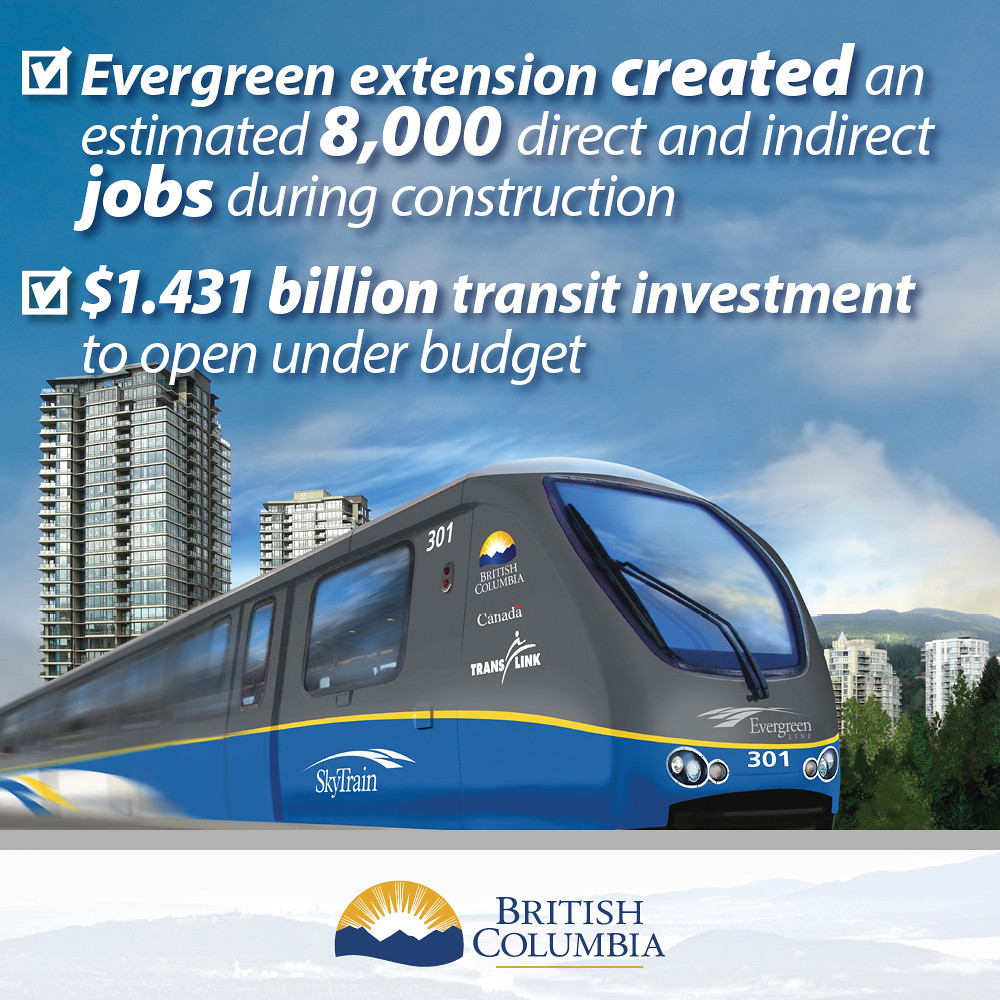The image features a rectangular advertisement for British Columbia showcasing the SkyTrain, prominently depicted in the center. The train is primarily gray with a blue lower half and a yellow strip in between. The train is heading from the left towards the right, with "301," "British Columbia," "Canada," "TransLink," and "SkyTrain" inscribed on its side. The front windshield reflects a partly cloudy sky and is labeled "Evergreen 301." Above the train, large white text on the blue sky background reads, "Evergreen Extension created an estimated 8,000 direct and indirect jobs during construction," followed by "1.431 billion transit investment to open under budget." To the left of the text are blue or white checkmarks for emphasis. In the backdrop, multi-story buildings dominate the left side, while additional high-rises and green trees can be seen further in the distance to the right. At the bottom, the words "British Columbia" are displayed in uppercase letters next to a sunset logo featuring yellow and blue colors and a mountain silhouette.